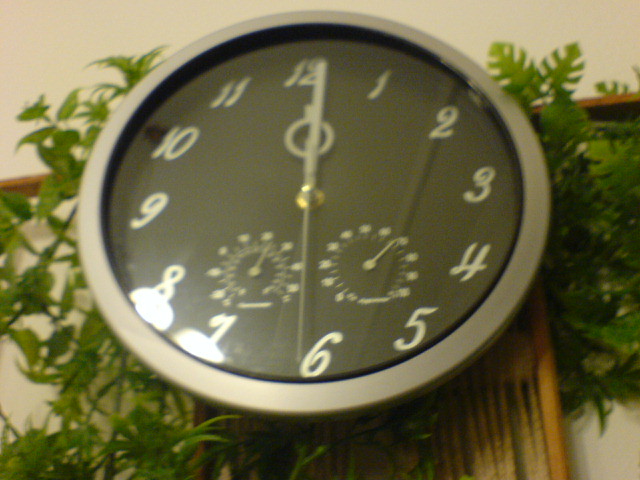The photograph captures a charcoal gray clock viewed from a slightly upward angle, creating an asymmetrical composition. The clock is either hanging or placed against a unique background featuring a blend of gray, pink, and green hues, adding an element of visual intrigue. A horizontal piece of wood in the background suggests it may be mounted, though this isn't immediately clear. The clock displays standard numerals from 1 to 12, with the hour and minute hands indicating the time as 12:30. Below, two smaller sub-dials add to the complexity of the design, though their exact functions remain uncertain. The overall setting and perspective evoke a sense of curiosity and contemplation.